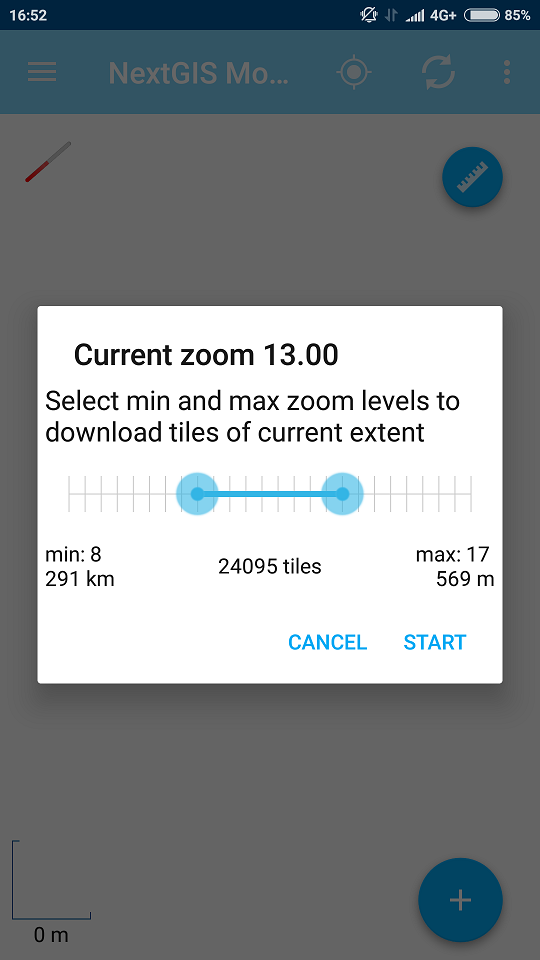This is a detailed screenshot from a smartphone display. At the top, a thin blue bar spans the width of the screen, displaying the time "16:52" (4:52 p.m.) in white text on the left. On the right, there is a circular blue icon followed by two stylized symbols: one resembling a vertical line with a leftward notch, and the other with a rightward notch at the top. Adjacent to these symbols is an icon denoting phone signal strength, represented by ascending bars. This is followed by "4G+" indicating the mobile network type, and a white battery icon displaying "85%".

Below the blue bar, the page features a two-inch thick blue section at the top, with a slightly dimmed blue background, likely due to a white pop-up box centered on the screen. The pop-up box is topped with the text "Current Zoom 13.00" in black. Below this, it reads, "Select min and max zoom levels to download tiles of current extent." There is a graphic resembling a train track, with a horizontal line intersected by a vertical bar. Two blue circles are connected by this line. 

On the left side, the text "Min, 8" is displayed, followed by "291KM" underneath. Centrally located, the pop-up shows "24095 tiles." To the right, it states "Max, 17" with "569M" below. At the bottom of this pop-up, beneath the "tiles" and "max" labels, there are two options: "Cancel" and "Start" in blue.

The dimmed background page features, in the bottom right corner, a blue circle with a white plus sign. On the blue bar above, white text reads "NextGISMO" followed by an ellipsis.